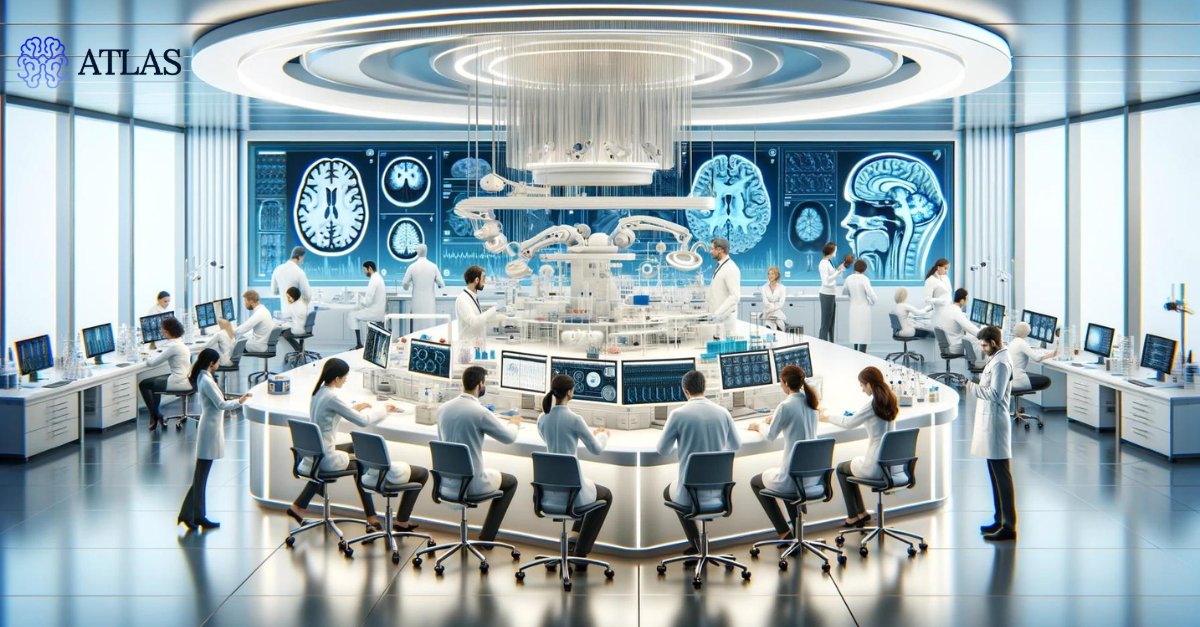This highly detailed digitally rendered image depicts the interior of a sophisticated scientific laboratory that appears almost photorealistic, possibly from a computer simulation or game. Central to the scene is a large, pristine white table that resembles a conference table, surrounded by seven scientists seated in high-backed chairs and two additional scientists standing. Each scientist is dressed in long lab coats over dark pants, engrossed in work at their computer monitors.

Above the table, a large white multi-armed device extends downwards, contributing to the high-tech ambiance. The floor is tiled, shiny, and impeccably clean. The room is illuminated by a large display in the background, showcasing detailed MRI or CT scans of the human brain and head in various sections, primarily in shades of blue and black. Prominently, the upper left-hand corner features a blue outline of a brain labeled “ATLAS” in bold, black uppercase letters.

Adding to the realism and complexity of the laboratory, additional desks with monitors line both sides of the room, with opaque glass windows behind them, possibly hinting at segregated workstations or additional observation areas. Despite its digital nature, the intricate details and scientific elements contribute to the convincing depiction of a bustling and advanced medical research facility.